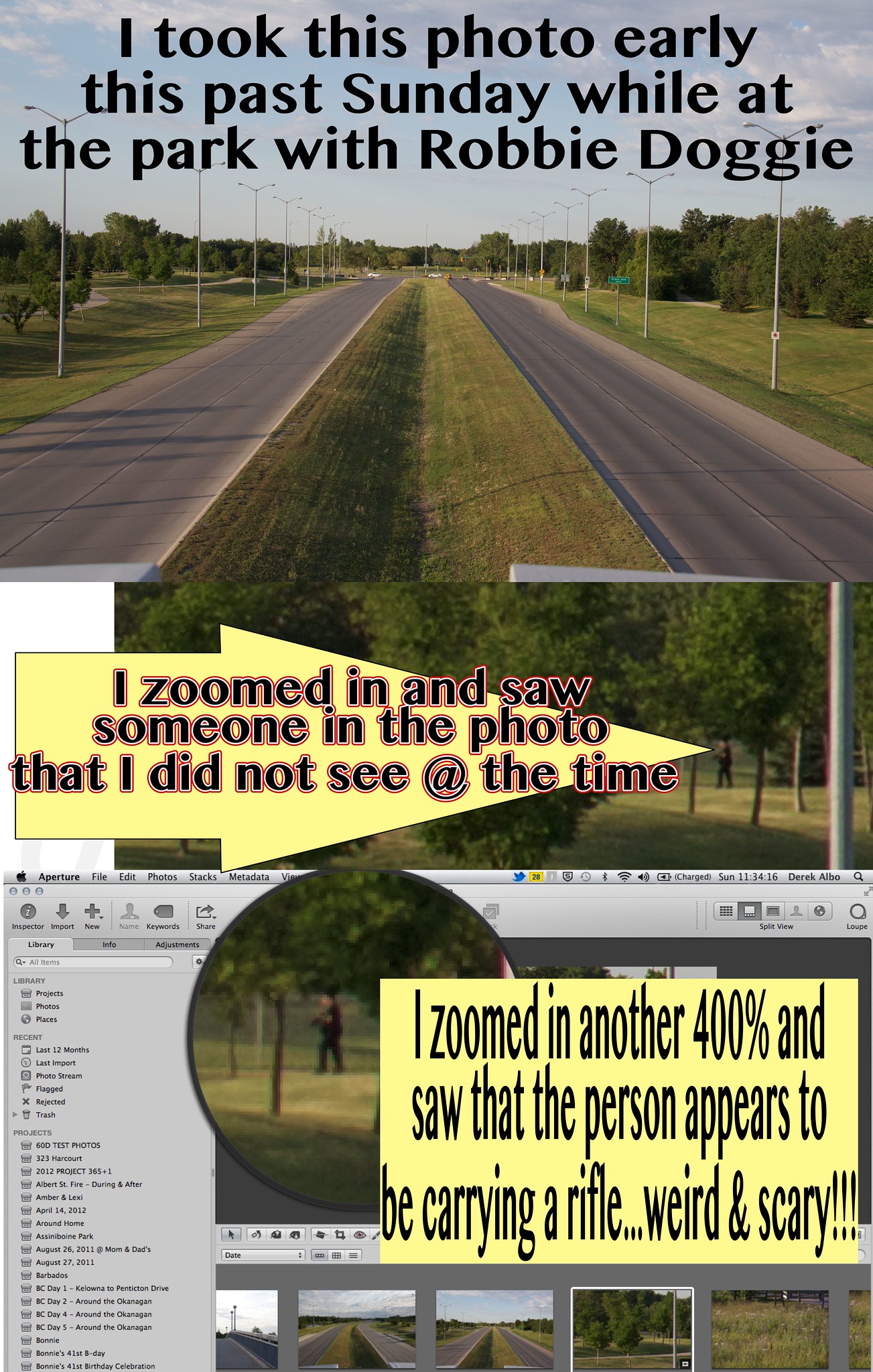The image is a collage of three photos shared on a computer screen, possibly for social media. The top photo, captured early this past Sunday, shows an outdoor scene from a park near a highway, with trees, a green space, and empty street lanes bordered by lamp posts. The accompanying text reads: "I took this photo early this past Sunday while at the park with Robby Doggy." 

Beneath it, there's a close-up of a shadowy figure amidst the trees with a yellow arrow pointing towards it. The inserted text says, "I zoomed in and saw someone in the photo that I did not see at the time." 

The bottom part of the collage is a screenshot of the same photo further zoomed in by 400%, with text in the yellow box stating, "I zoomed in another 400% and saw that the person appears to be carrying a rifle, weird and scary!!!" The figure, dressed in dark clothing, appears to be holding something over their arm, though it's unclear if it's actually a rifle.